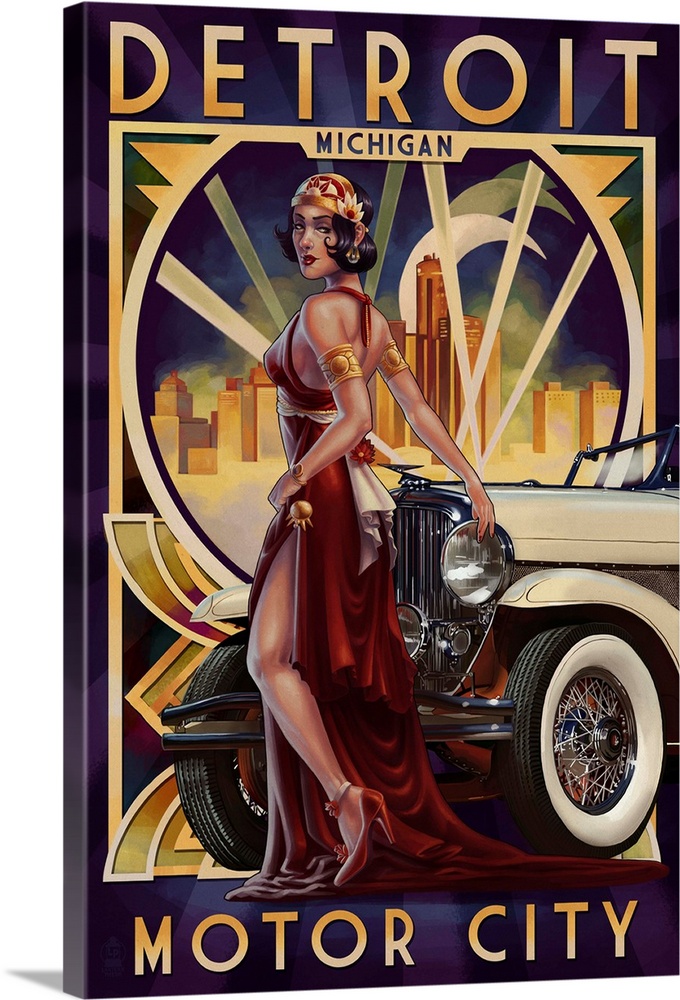This digitally created rectangular canvas print depicts a stylish woman embodying the glamorous fashion of the 1930s or 1940s. She wears a slinky, scarlet red dress with a thigh-high slit and matching red high heels. Adorned with golden cuffs on her upper arms, long earrings, and a partial scarf on her head, she stands confidently posing in front of a vintage white car, likely from the 1920s or 1930s, which features classic headlights, a grill, and thin, white wall tires. Her left hand rests lightly on one of the headlights, while she glances over her left shoulder. The background showcases a golden cityscape, illuminated by spotlights that accentuate the era’s Art Deco style. The text "Detroit Motor City" is prominently displayed, with "Detroit" at the top in yellow, "Motor City" at the bottom, and "Michigan" in smaller blue text beneath "Detroit." The overall vibe is reminiscent of a throwback advertisement celebrating the iconic automotive heritage and glitz of Detroit.